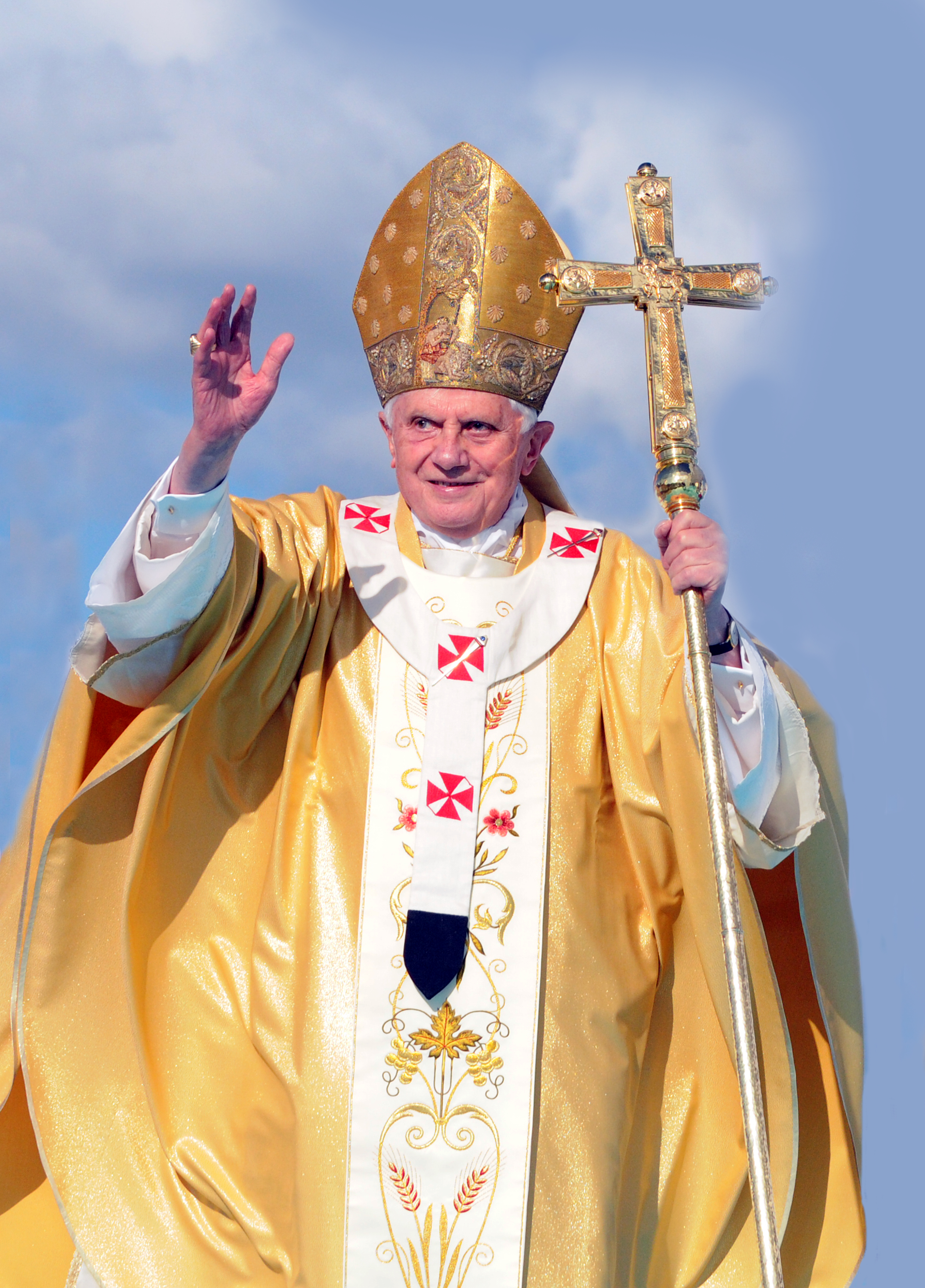In this detailed image, we see an elderly Pope, likely Pope Francis, dressed in elaborate papal regalia. He has deep-set eyes and short gray hair peeking from beneath a towering, gold embellished miter hat which is almost diamond-shaped, adorned with intricate floral and cross designs. Pope Francis is wearing a striking yellowish-gold robe that features multiple crosses and elaborate gold and red embroidery. Beneath this robe, several layers of white attire are visible, including a white collared shirt and a poncho-like garment, suggesting he is clad in numerous ceremonial layers.

In his left hand, he holds a long silver staff topped with a thick, ornate gold cross that matches the color and intricate design of his headpiece. His right hand is raised in a gesture that suggests greeting or blessing. A gold ring is also noticeable on one of his fingers. The background shows a serene blue sky with a few wispy white clouds, adding a tranquil aura to the image. Pope Francis looks serene, with a slight smile on his face, embodying both the solemnity and grace of his office.